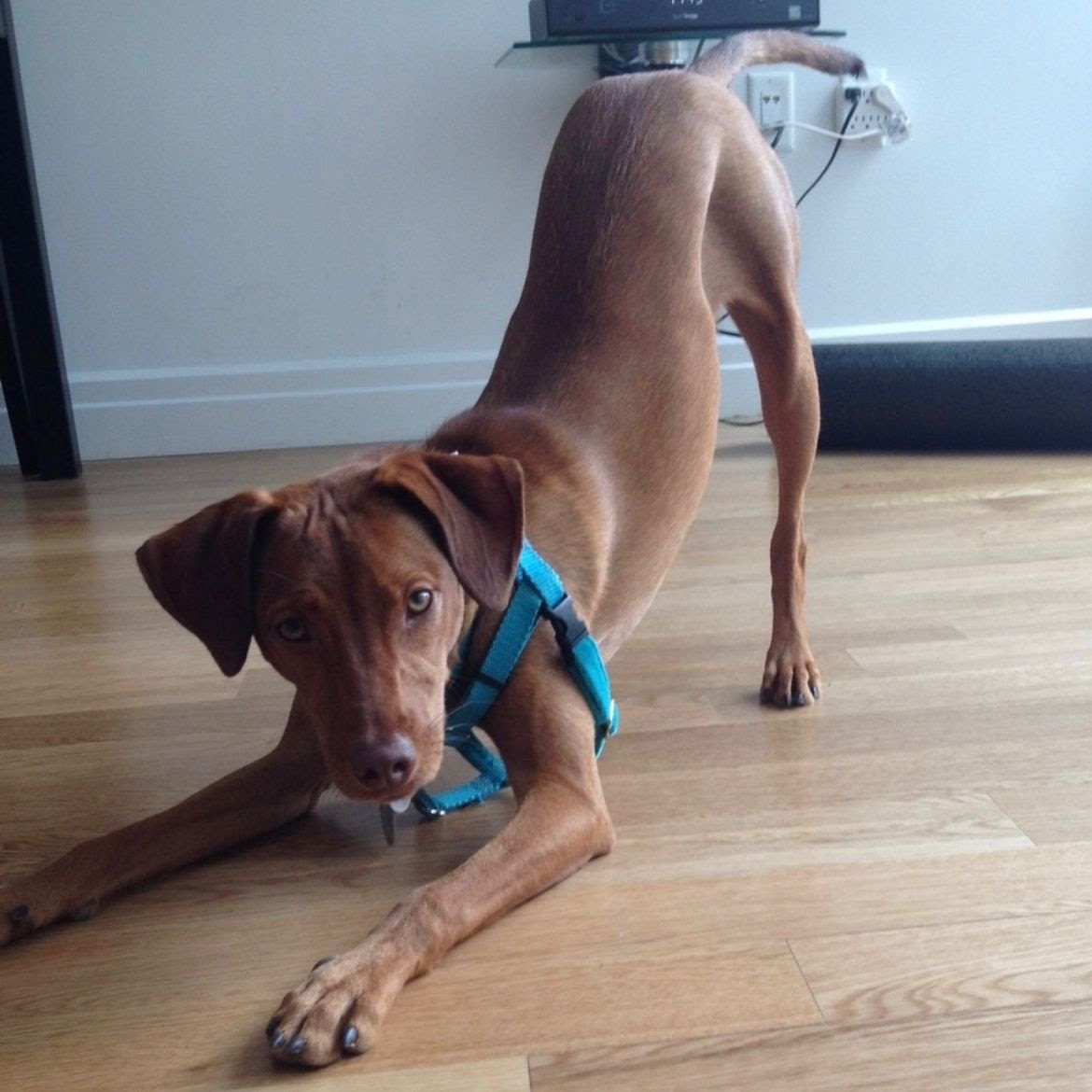This image depicts a light caramel brown dog in a serene downward dog yoga pose, showcasing its arched back and extended front legs. The dog is adorned in a turquoise-blue harness, giving a pop of color against the predominantly brown scene. Captured indoors with a phone camera, the setting features a hardwood floor of a light almond hue that complements the dog's coat. In the background, there's a white wall with multiple electrical outlets, where various devices are plugged in. To the right side of the image, a black object resembling a pillow is visible, while to the left, part of a table or dresser leg is seen. The dog's expression is peaceful and neutral, as it gazes directly at the camera, almost as if posing for a photo or a competition.